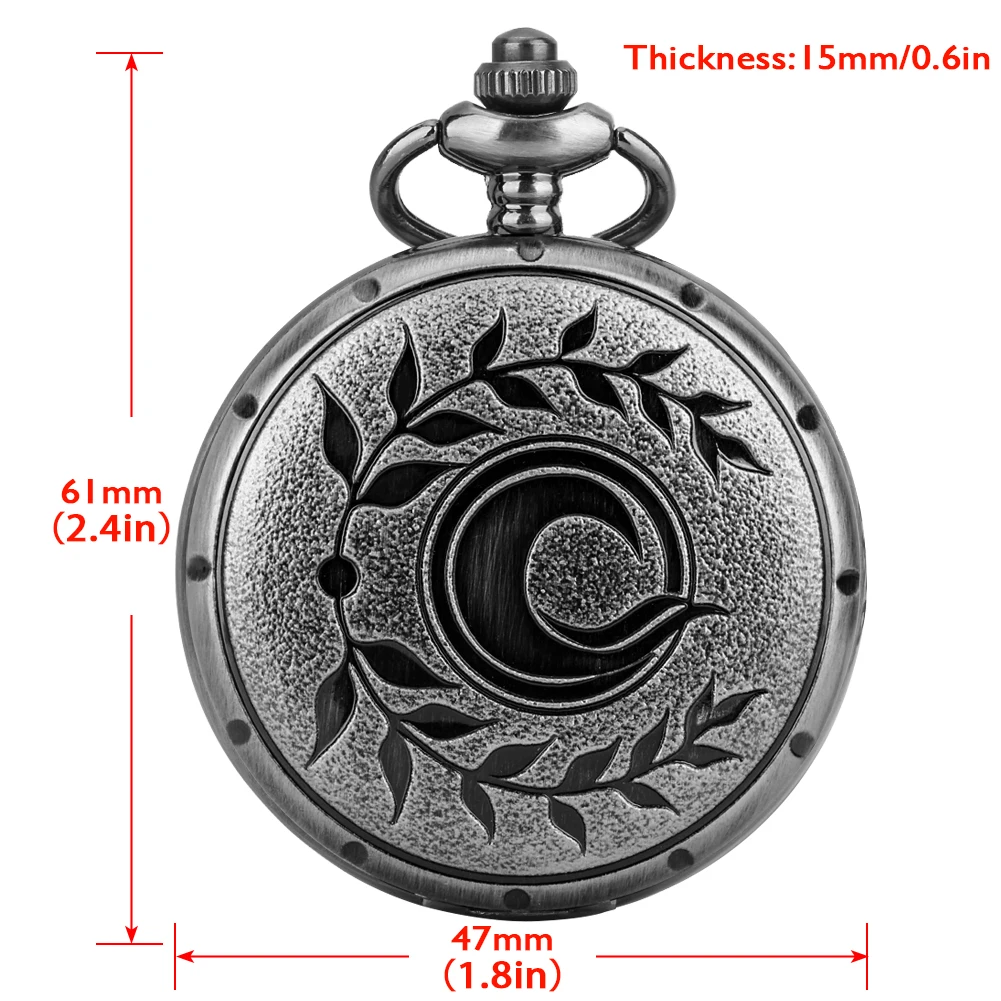Close-up rendering of the back of a pocket watch, depicted in shades of gray. The pocket watch has a silver hue with a dark textured finish and features a black vine design with leaves encircling the edge. The rim of the watch is smooth, adorned with 12 small, dark circular indentations evenly spaced around it. Accompanying the image is red text indicating the dimensions of the watch, as well as thin red arrows. At the top, the text reads "Thickness: 15 millimeters (0.6 inches)" with an arrow pointing vertically. In the middle, horizontal arrows mark the width and height, labeled "61 millimeters (2.4 inches)" and "47 millimeters (1.8 inches)" respectively.